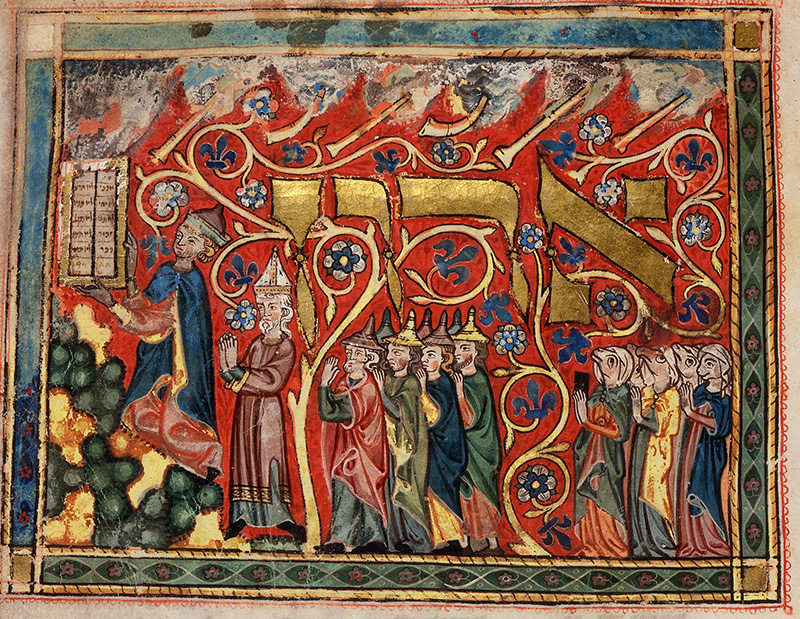This image appears to be a detailed and ancient mural or tapestry, possibly a thousand years old, depicting a religious procession. The central figure on the left side of the scene is a man in a blue robe, holding aloft a framed scripture or parchment with gold writing. He is slightly elevated and is not facing the procession, which moves to the left. Behind him, there is another prominent religious figure dressed in robes and wearing a pointed hat, possibly a bishop, who seems to be praying.

Following these two figures are several people, all in variously colored conical hats and robes of red, blue, and green. These individuals are depicted in a prayerful stance as well. In the background, mainly on the right side, stand figures that appear female, identifiable by the outlines of their breasts visible under their dresses. However, these women have goat-like heads with slightly human features, presenting an otherworldly aspect to the procession.

The procession is set against a reddish background adorned with thin, trumpet-like gold figurines. The entire scene is framed by a decorative green border featuring elliptical shapes with red flowers at their centers, adding to the intricate details of this fascinating and mysterious artwork.